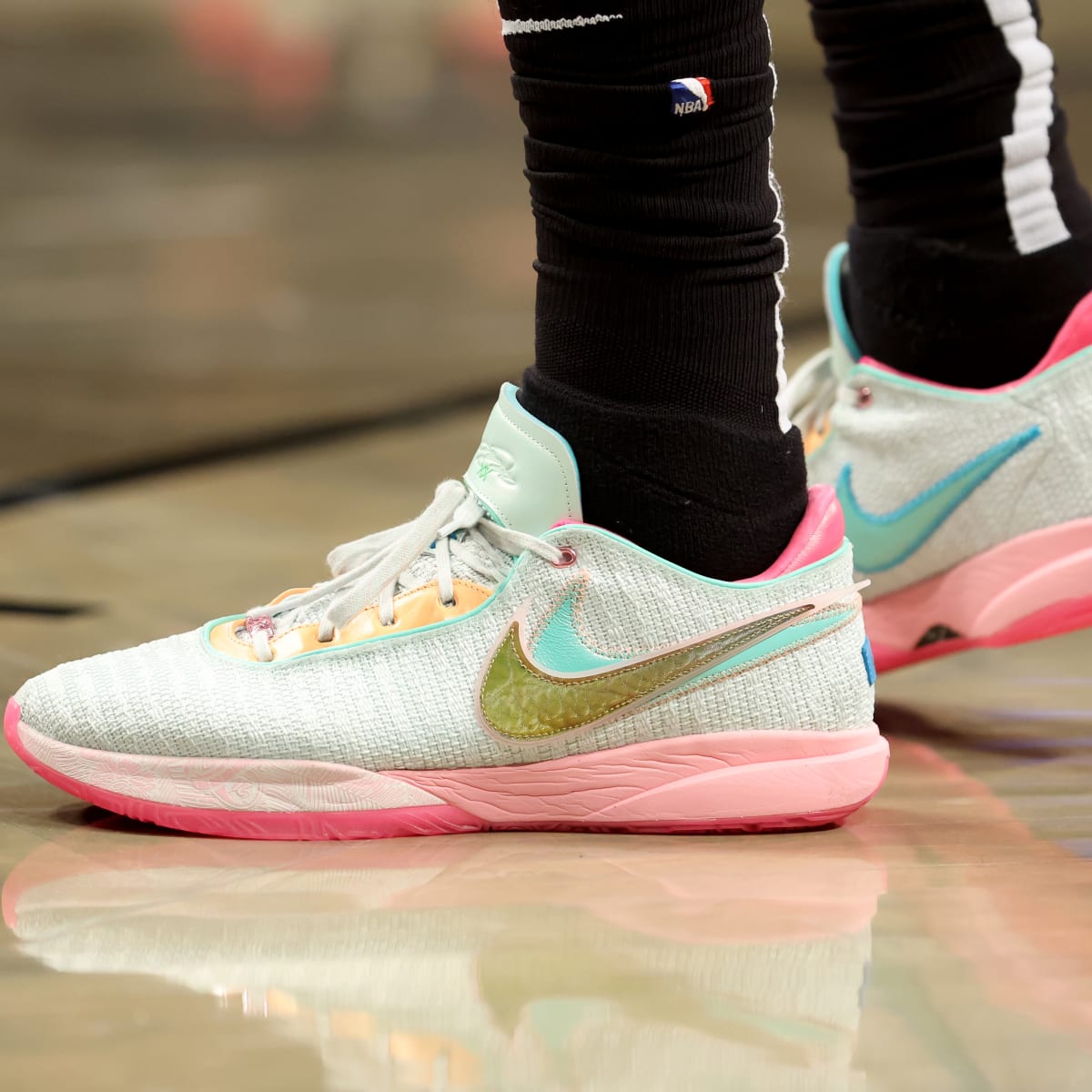The image is a detailed photograph of a woman’s new Nike sneakers taken on a shiny hardwood basketball court. The sneakers are predominantly white with pink soles, white laces, and feature a Nike swoosh. One shoe presents an olive green swoosh overlapping a teal blue swoosh, while the other has a simple teal swoosh. The photograph captures only the woman's ankles and feet, leaving the rest of her body cropped out. She is wearing black socks adorned with a wrinkled NBA logo that includes blue, white, and red accents, as well as a white line at the back of the socks. The setting highlights the glossy hardwood floor, suggesting a basketball court, and the position of her feet in the center with one foot more prominently in the foreground. The image is likely intended to showcase the stylish new Nikes in an NBA-related context, emphasized by the visible reflections on the polished court and the distinct combination of colors like pink, greenish-blue, lime, and baby orange in the design of the shoes.